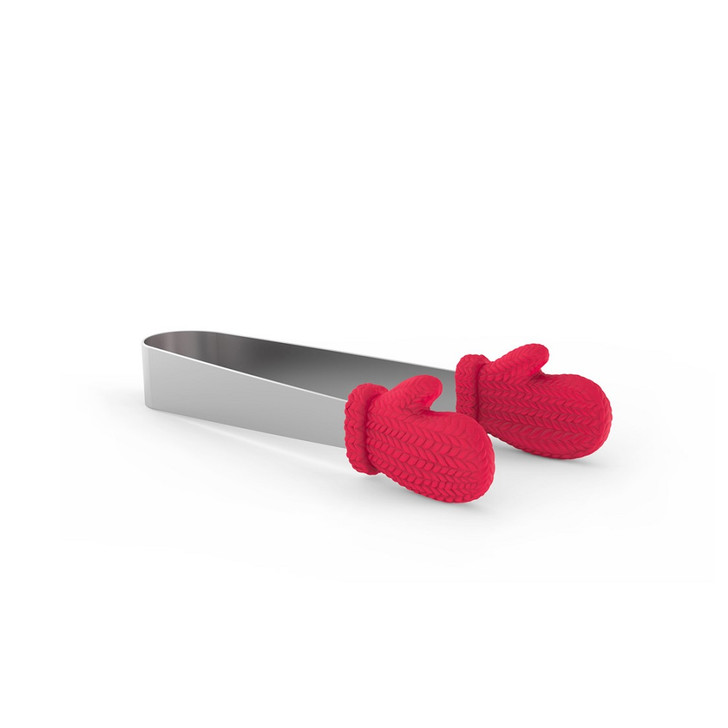This image features a pair of silver food tongs against a completely white background. The striking detail of the tongs is the attachment at the gripping end: two crocheted red mittens, complete with cuffs, resembling tiny oven mitts. The mittens have a distinctive knitted appearance, suggesting a homespun touch, and feature a design akin to tire tracks, providing texture. The image appears minimalistic, with only a faint shadow to suggest depth, likely intended for online presentation or sale.